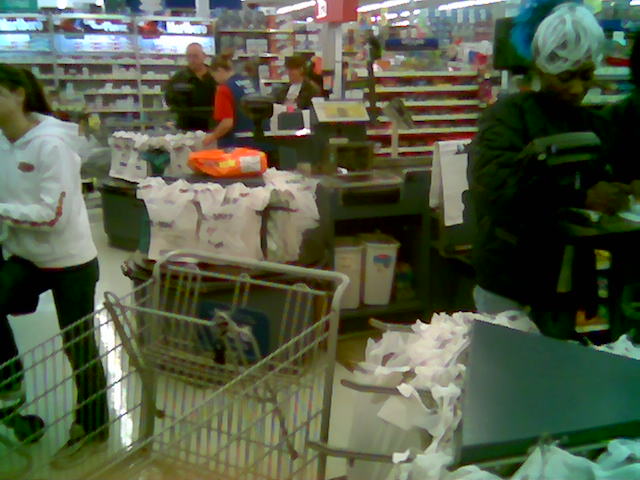This photograph, capturing an older scene inside a supermarket, focuses on the checkout aisles. One can see a rotating circular device filled with numerous plastic bags and a register equipped with a conveyor belt. At the checkout closest to the viewer, an African-American woman with white hair is writing a check, while nearby, a Caucasian woman in a white jacket and black pants, or possibly a white jumper and blue jeans, stands with a shopping cart. Notably, another shopping cart in the foreground is gray in color. Further back, the final register features a cashier wearing a red T-shirt with a blue vest, assisting a man and woman in line. Shelves filled with candy and a prominent advertisement for Marlboro cigarettes line the wall, enhancing the nostalgic feel of the supermarket.